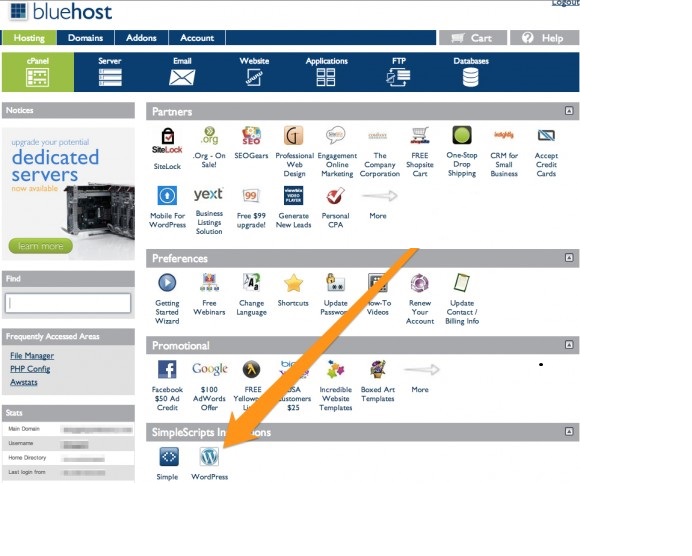Caption: 
The Bluehost dashboard features a detailed user interface. At the top left, the "Bluehost" logo is displayed in blue, while the top right corner provides a "Logout" option. Below these, a blue navigation bar prominently displays "Hosting" in green, alongside links for "Domains," "Add-ons," and "Account." To the far right of this bar are two gray buttons labeled "Cart" and "Help."

Further down, another blue bar lists essential tools in green, including "cPanel," with adjacent links for "Server," "Email," "Website," "Applications," "FTP," and "Databases," each accompanied by intuitive icons.

Under the "Partners" section, various services are listed, such as SiteLock, SEO Gears, Professional Web Design, Online Marketing, and many others tailored for diverse business needs. Each service is represented with corresponding icons.

On the right side, an orange arrow points to a WordPress icon, partially obscuring the "Simple Scripts" section. Meanwhile, a promotional ad on the left encourages users to upgrade to dedicated servers, featuring a server image and a green "Learn More" button.